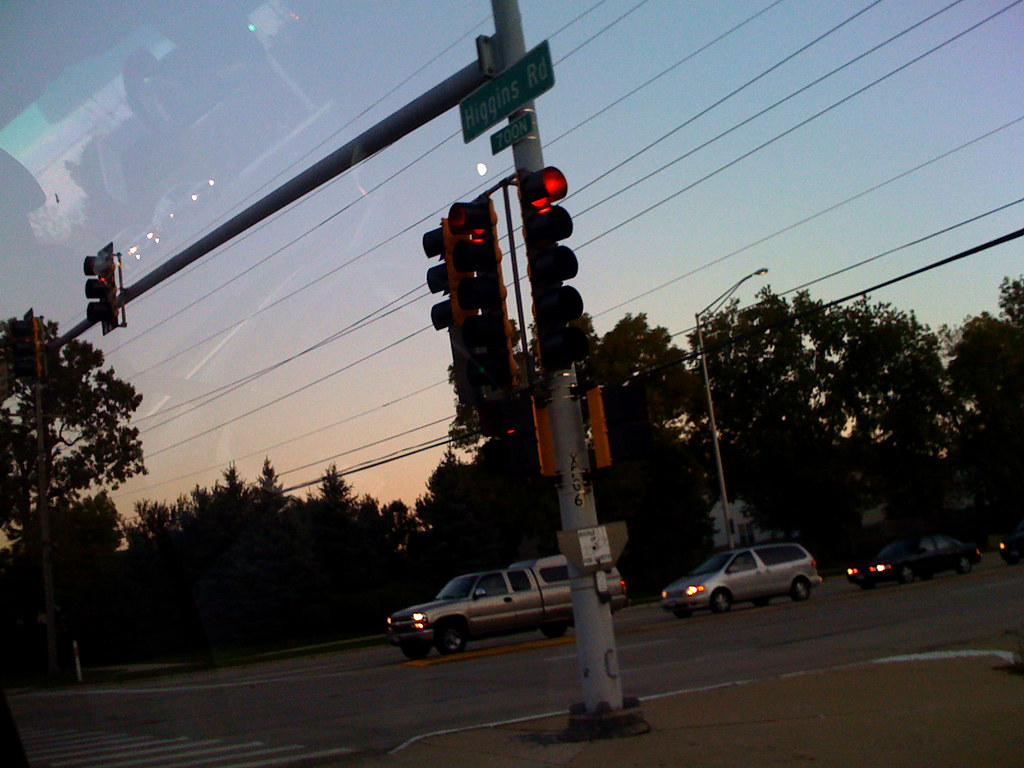The image captures a view through a car window, evident from the reflection in the upper left-hand corner. The scene reveals a dusk-lit intersection with a gray-blue sky fading into a pinkish-orange near the horizon. Prominently in the frame, there is a traffic light assembly featuring a single pole with both vertical and horizontal arms, each fitted with red-lit traffic lights. Below the suspended lights, three vehicles—a pickup truck, a minivan, and a sedan—are stopped, their headlights casting beams on the predominantly gray street, which is lined with white markings and a touch of yellow paint. Trees loom darkly in the background, while an array of overhead power lines and streetlights add complexity to the scene. A green street sign labeled "Higgins Road" with an unreadable smaller green sign beneath it is attached to the light pole, standing on light brown ground. The lighting, with sun setting behind, casts everything in shadow, reinforcing the time of day as early evening.